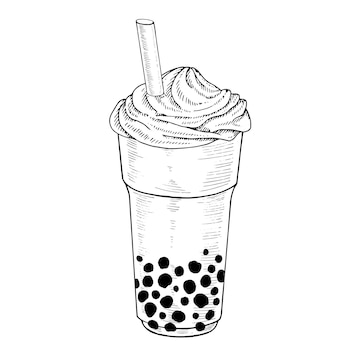This black and white, hand-drawn image depicts a distinctive cup that appears to be a hybrid of a milkshake and a bubble tea. The 16-ounce white Styrofoam cup is detailed in stark black ink or pencil lines and is adorned with black polka dots of varying sizes covering approximately the bottom third of the cup. Rising from the whipped cream topping, which is illustrated with textured ridges like a small conical volcano, is a large-diameter plastic straw positioned to the left. The base of the cup is filled with what appear to be boba pearls, reinforcing the impression of a bubble tea fusion. The drawing features no text or lettering, and the entire scene is set against a plain white background.